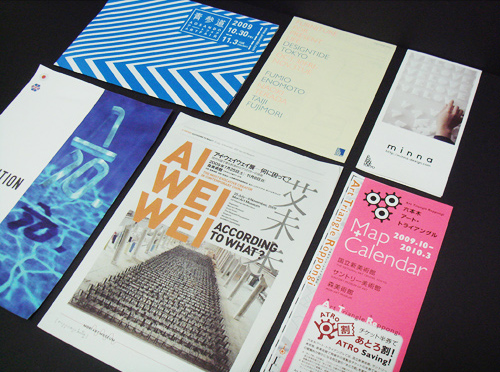The image shows an assortment of flyers and pamphlets neatly organized in two rows on a black background surface. In the top left corner, there is a card with blue, arrow-like lines and Chinese characters, with the dates "2009, 10.30, 11.3" noted on the top right. Next to it, there is a white rectangular flyer titled "Design Tide Tokyo" with names like "Fumio" and "Taji Fujimori" written on it. To its right lies a smaller white card labeled "MINA" featuring an image of a hand. 

In the bottom row on the left, there's a flyer divided into two halves; one side has a white background and the other depicts an underwater scene, though the writing on it is indistinguishable. The next flyer to the right has a white background with an image of several rows of chairs at the top. It contains the text "Ai Weiwei, According to what." Lastly, on the far right, there's a pink flyer that states "Map + Calendar, 2009.10 - 2010.3."